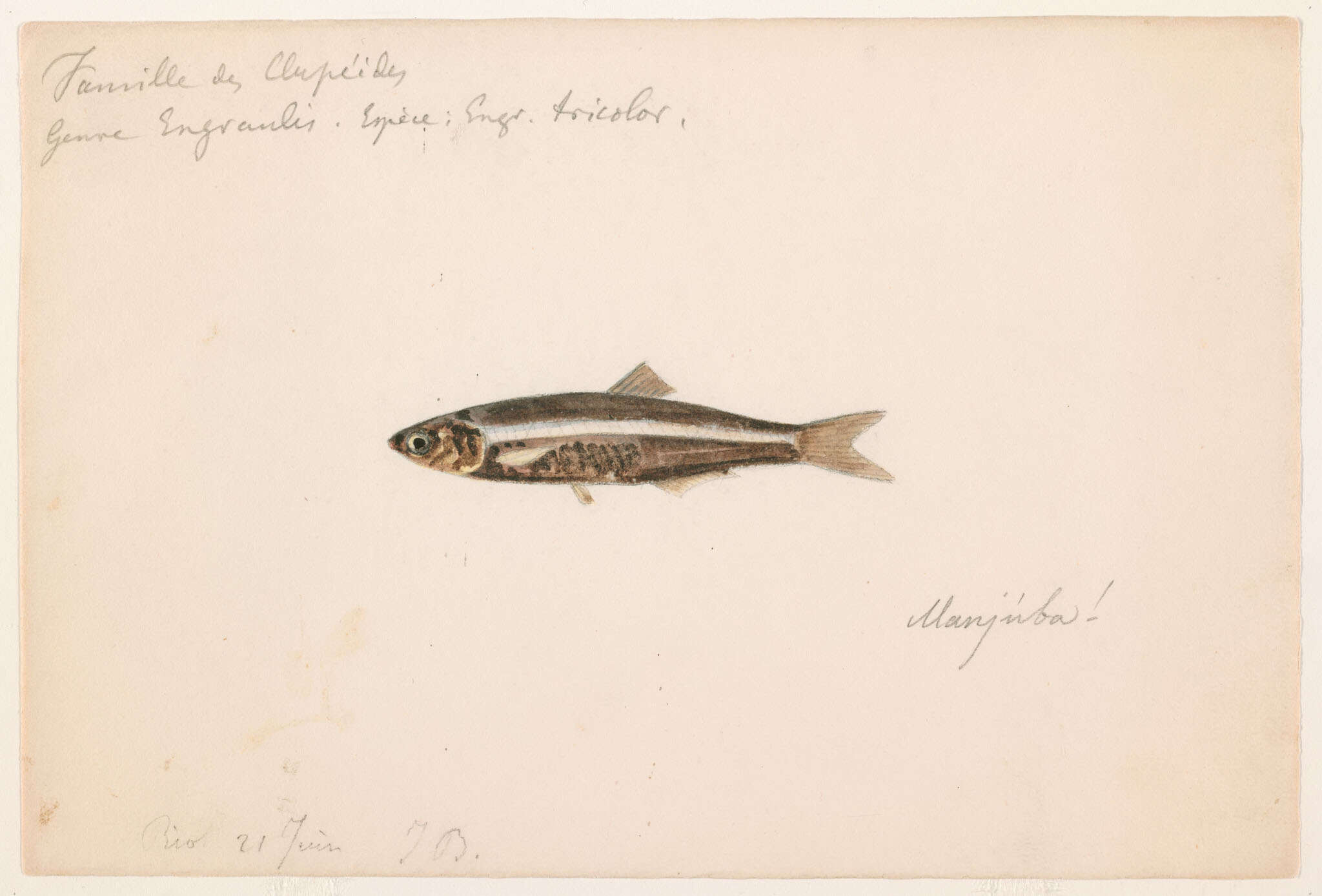This image depicts an old, rectangular illustration or print of a small fish, likely an extinct or rare species given the detailed presentation. The paper is aged to a beige color with darker brown stains and marks, giving it an antique appearance. It is bordered by a white edge, suggesting a mounted display.

At the very top of the image, there's cursive handwriting, difficult to decipher but possibly indicating the fish's species name. The only legible English word is "tricolour," likely referring to the fish's coloring. Handwritten notes are also visible in the lower left and right corners of the illustration.

The fish itself is narrow and small, resembling a sardine with an elongated, surfboard-like shape. It has a small, pointy head with a notable golden eye featuring a black pupil. The head is brownish, and its body showcases a pronounced white stripe running along the side. The top spine area is dark brown, while the rest of the body transitions into browns and silvers. The fish has small, light brown fins and a light brown tail, adding to its delicate appearance.